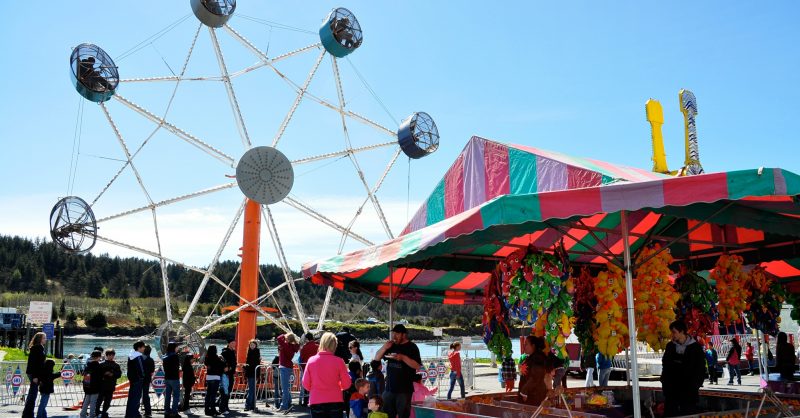The image captures a bustling fair scene, set against a backdrop of a clear blue sky and a serene lake surrounded by a natural forest. On the right side, there's a large canopy area with a circus tent-like top adorned in vibrant Easter colors of purple, teal, and pink. Underneath the canopy, which is set up like a carnival game stall, a variety of yellow and green stuffed animals are hanging as prizes, with people gathered around, presumably trying their luck at the games.

To the left, crowds of people are seen waiting to board a small Ferris wheel. This Ferris wheel features an orange steel beam structure and is equipped with small, snowflake-shaped cages that look like they can hold one person each. The ride is encircled by silver guardrails, adding to the safety and organization of the fairground. The bottom portion of the image is lively with numerous visitors walking around, enjoying the festive atmosphere under the bright and clear daylight.